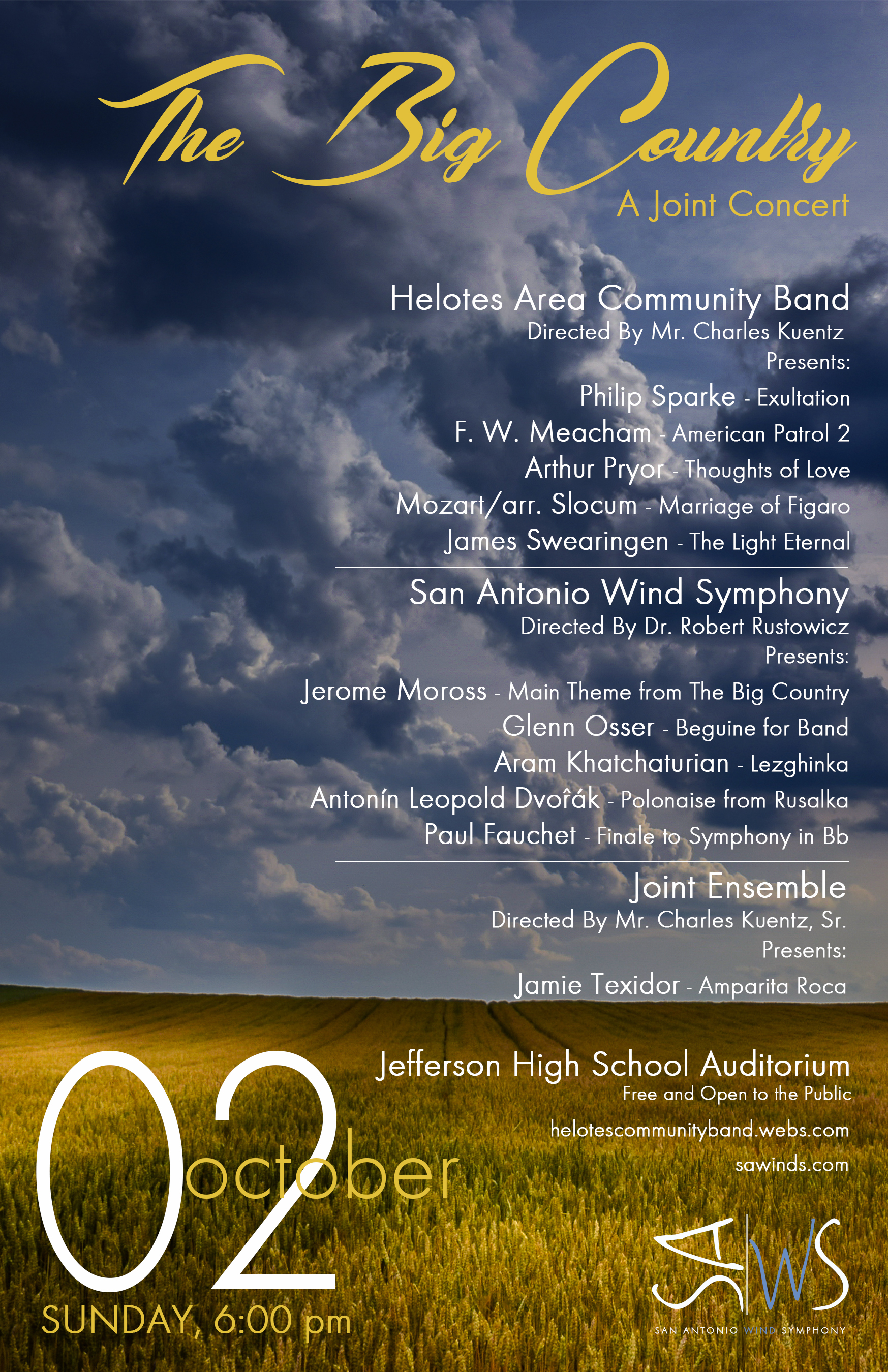This vibrant color advertisement promotes an upcoming concert. The background ambiance is set by a stormy, heavily overcast sky, beneath which lies a serene field of yellowish-green grass. Roses dot the landscape, beginning from the middle of the image and extending outward. 

In elegant yellow script at the forefront, the title "The Big Country" is displayed. Below it, in plain text, is a detailed rundown of the concert's participants and pieces. The H-E-L-O-T-E-S Area Community Band, directed by Mr. Charles Kuentz, will present:

- Phil Sparke's "Exaltation"
- F. W. Meacham's "American Patrol II"
- Arthur Pryor's "Thoughts of Love"
- Mozart (arranged by Slocum) with "Marriage of Figaro"
- James Swearengin's "The Light Eternal"

Following them, the San Antonio Wind Symphony, under the direction of Dr. Robert Rustowicz, will feature:

- Jerome Moross's "Main Theme from The Big Country"
- Glenn Osser's "Beguine for Band"
- Aram Khachaturian's "Lezginka"
- Antonín Dvořák's "Polonaise from Rusalka"
- Paul Fauchet's "Finale to Symphony in B-Flat Major"

A joint ensemble, directed by Mr. Charles Kuentz, Sr., will culminate the event with Jaime Texidor’s "Amparito Roca."

The Jefferson High School Auditorium opens its doors for this free event, welcoming everyone to join at 6 p.m. on Sunday, October 2nd. Detailed information, including community band resources, can be found at helotescommunityband.webs.com and sawinds.com. In large letters at the image's bottom right corner is "San Antonio Wind Symphony."